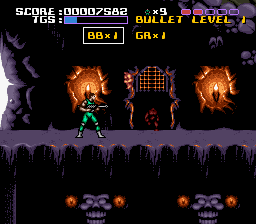This screenshot captures the essence of a vintage video game, potentially from an older console or a mobile device, characterized by its low-resolution graphics. Dominating the lower third of the image is a dark gray, almost purplish, fence. In front of this fence, two glowing skulls are prominently placed, each flanked by candles on either side, adding an eerie illumination.

Above the fence, there is a visible walkway. On this path stands a figure dressed in a green outfit, armed with a rifle or a similar firearm. The surroundings suggest he is inside a cave, identifiable by a few alcoves on the cave walls that hold additional candles, casting dim light around the space.

Centrally positioned in the background is a metal door with small holes, allowing light to peek through, adding to the sense of mystery. The top section of the screen displays conventional game metrics such as the score, remaining bullet count, and lives left—further emphasizing its classic game design.

An intriguing detail is the left edge of the screenshot, which appears to be peeled away, suggesting either an intentional artistic choice or damage to the image, enhancing its nostalgic and worn-out appeal.